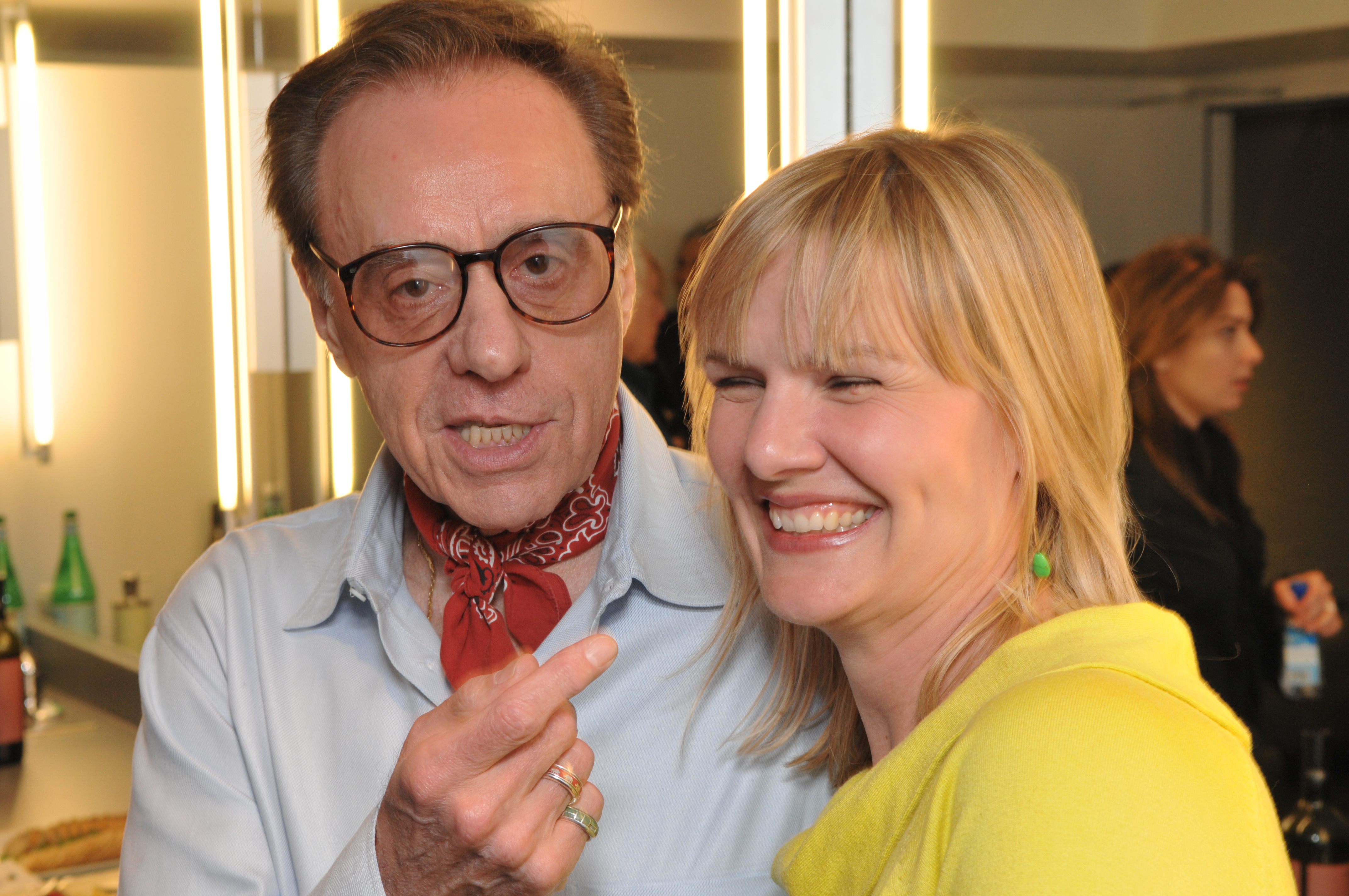The photograph is a horizontally aligned rectangle, with two Caucasian individuals, both appearing to be in their early 50s, standing side by side. Positioned slightly to the right of the center, the man and woman are both active-looking and in good shape. The man has short, possibly dyed red hair with a receding hairline. He wears glasses and a red kerchief tied around his neck over a pale blue collared, long-sleeved shirt. He has silver rings on his pinky and ring finger of his right hand, which is pointing toward the woman next to him. He has a half-smile on his face as he looks slightly left and down.

The woman next to him has long, straight, glossy blonde hair that’s styled either in a gentle mullet cut or a stylish braid. She is grinning broadly, her eyes are squinting, and she appears to be laughing, showcasing her teeth. She adorns green dangly earrings and wears a bright yellow smock top shirt. She stands slightly shorter than the man and holds a blue-topped water bottle.

In the background are vertical tubes of fluorescent lights and a mirror on the left side reflecting a green glass bottle with yellowish liquid and a brown bottle with a pink label. Above the mirror is one of the vertical lights, while the other two lights appear closer to each other with a window between them. Below the bottles is a peach-colored surface with a brass or gold border. Between the heads of the two main subjects, there is a reflection or a view through a window showing two individuals in black. The wall behind the window is mustard-colored, transitioning to white towards the right side, where there is also a doorway near the woman. 

The style of the individuals' clothing suggests influences ranging from modern to potentially retro, such as the man’s kerchief that hints at a 1970s style.